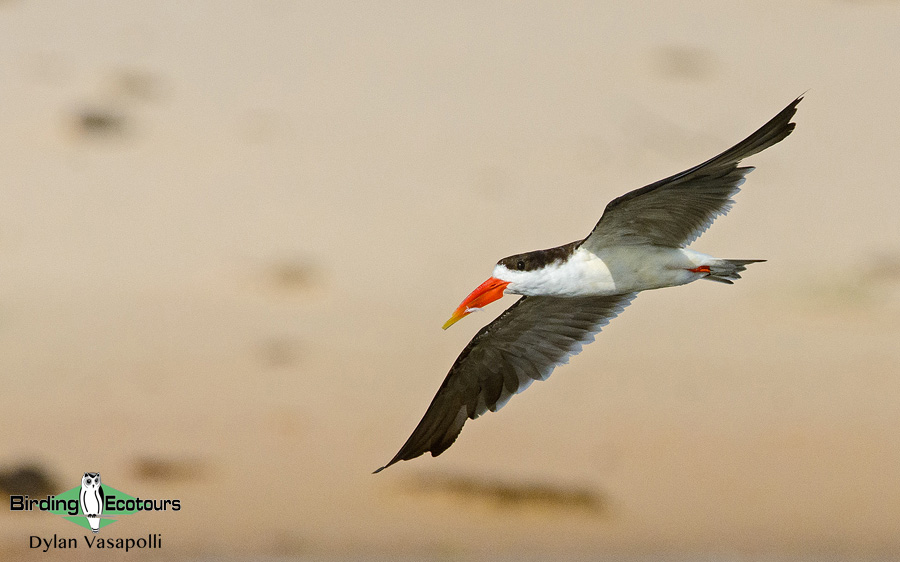This image captures a close-up of a bird in mid-flight, with its wings asymmetrically positioned—one wing is dipping lower than the other, suggesting a turning maneuver. The bird features a striking contrast between the black and white coloration: a white body, black wings with gray tips, and a black face. It has a distinct long orange bill with a yellow tip and orange feet tucked up against its body. The background is a blurred mix of tan shades and dark spots, possibly suggesting water with rocks or perhaps a gray sky with indistinct objects. In the bottom left corner of the image, there is a logo comprising the word "Birding" on the left, an artwork of a white bird in the middle, and "Ecotours" on the right side, followed by the name "Dillon Vasopoli" underneath.